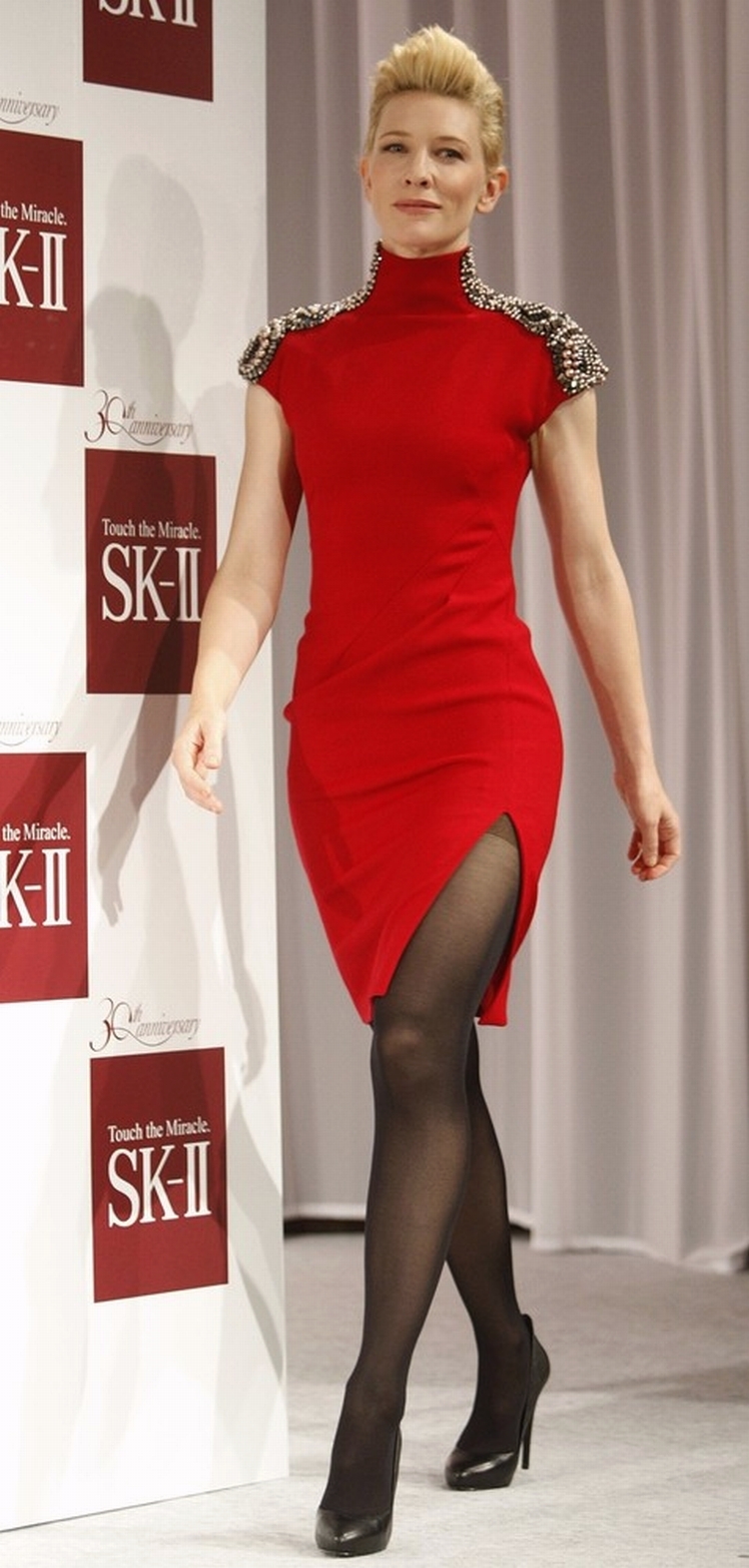In this photo, we see Cate Blanchett, a renowned celebrity, elegantly stepping onto a stage or photography set. She is wearing a striking red form-fitting dress featuring a slit up the left side. The dress is adorned with a turtleneck-like collar studded with white and black gems and pearls extending down to the short sleeves, adding a touch of sophistication and glamour. She completes her outfit with black stockings and black pump heels. Cate Blanchett's short blonde hair is stylishly combed up, adding to her poised appearance. The backdrop includes long white drapes and a distinctive wall to her side with red squares. The wall bears the words "Touch the Miracle," prominently featuring the SK-2 branding.